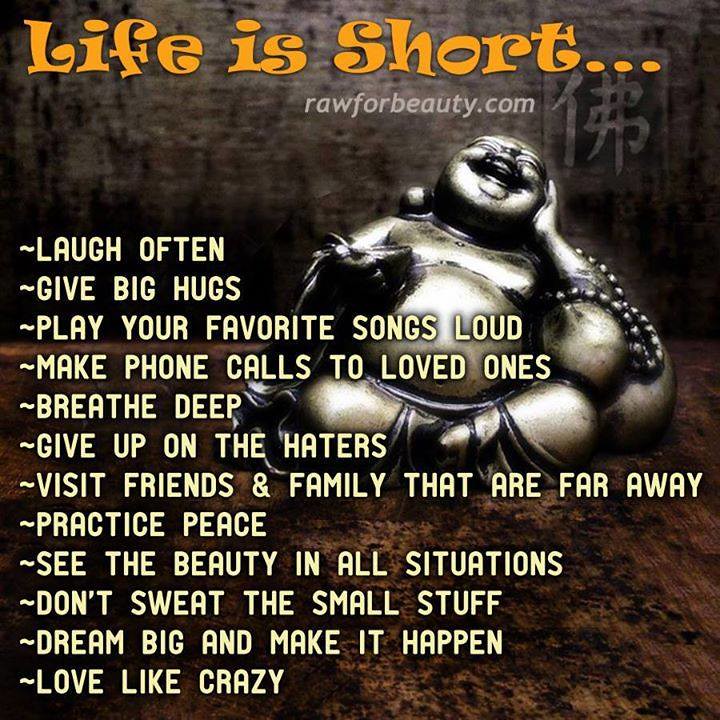The image is a colorful flyer with a motivational theme. Dominating the design is a serene, laughing Buddha statue, sitting cross-legged with one hand resting on his cheek and the other holding a bowl. The background of the flyer features subtle tones of brown and gray, with a faint Asian character in a square.

At the top, bold orange text declares, "Life is short..." followed by a series of life advice points listed in transparent white print next to squiggle-like bullet points. The advice includes: "Laugh often, give big hugs, play your favorite songs loud, make phone calls to loved ones, breathe deep, give up on the haters, visit friends and family that are far away, practice peace, see the beauty in all situations, don't sweat the small stuff, dream big and make it happen, and love like crazy." At the bottom of the flyer, the website "rawforbeauty.com" is printed in gray.